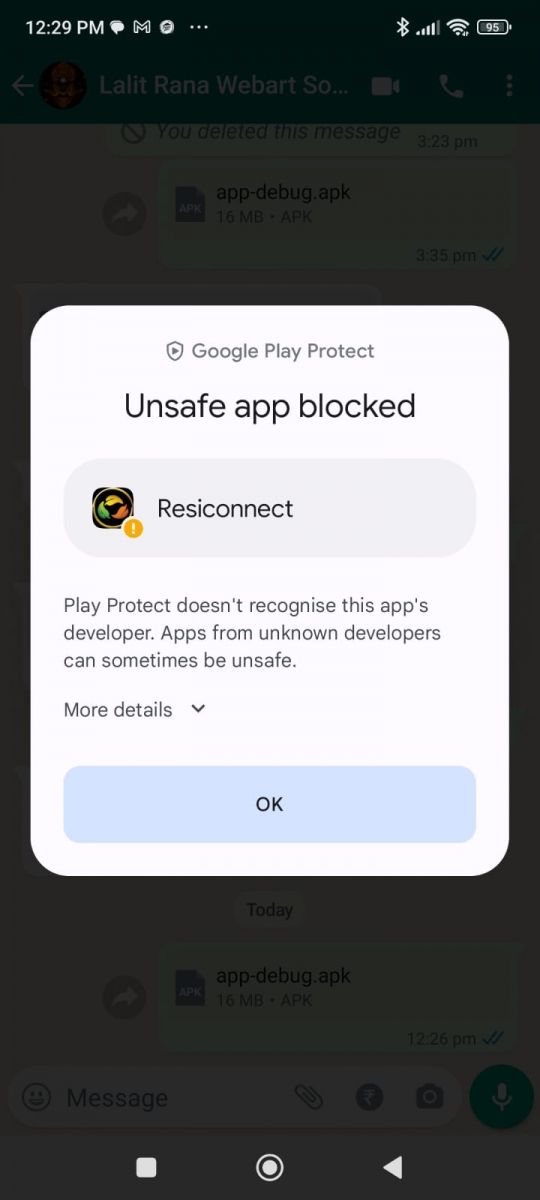The image depicts a smartphone screen in portrait mode. In the top left corner, the time is displayed as 12:29 p.m., alongside an envelope icon and a speech bubble icon. The top right corner shows additional icons: Bluetooth, reception strength, Wi-Fi status, and the battery icon indicating 95% charge.

Dominating the screen is a white pop-up notification from "Google Play Protect." At the top of the notification, bold black text reads "Unsafe app blocked." Below this, there's an app named "re rest rest I connect" with an icon featuring yellow, green, and orange leaf-like figures arranged in a circle, along with a yellow exclamation point signifying caution.

The notification further explains, "Play Protect doesn't recognize this app's developer. Apps from unknown developers can sometimes be unsafe." Beneath this warning, there's a blue button labeled "OK" and an option for "More details."

In the background, partially obscured by the pop-up, is a blacked-out section with a green header showing the name "Rena Weber." Below this header appears a series of text messages, one of which contains "app-debug.apk."